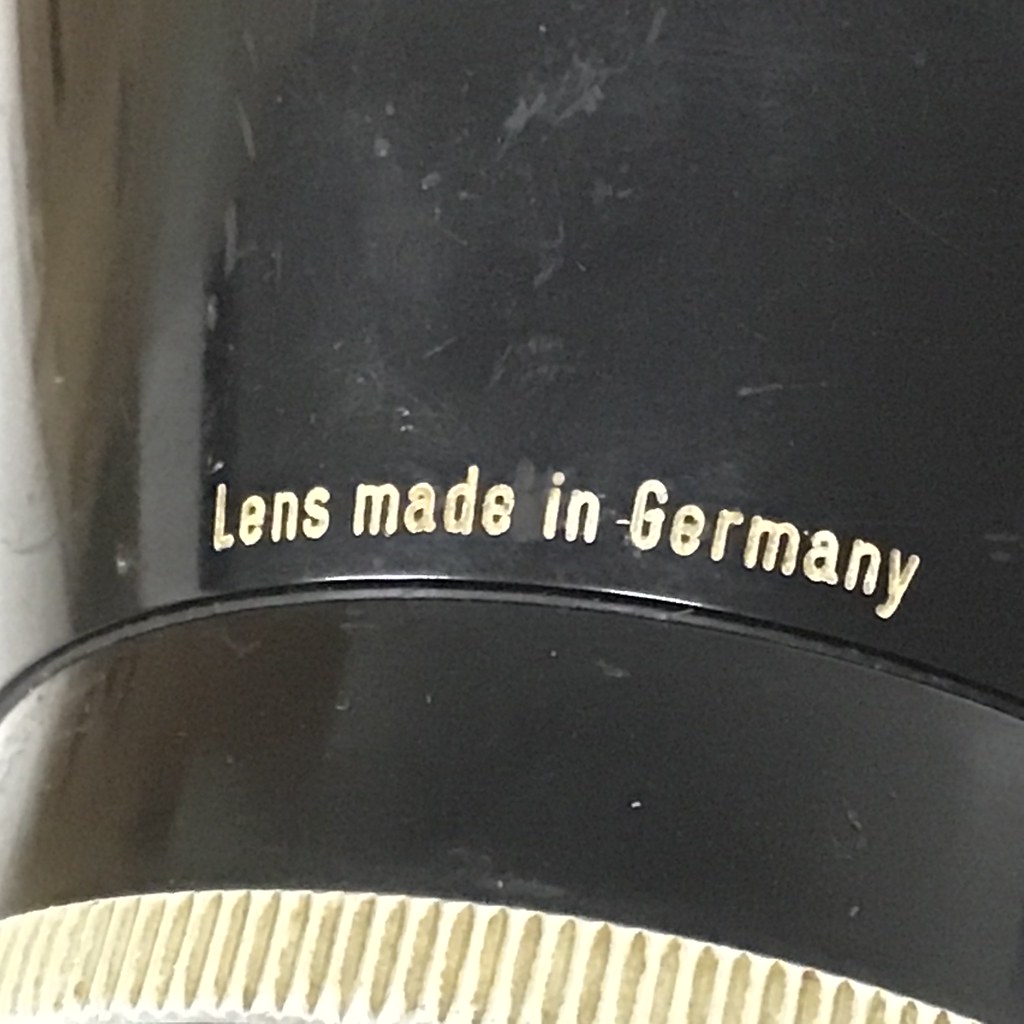This is a detailed close-up of a camera lens captured in a color photograph. The main focus is the black, shiny body of the lens, which exhibits a few subtle scuff marks showcasing its use. At the bottom edge, the lens has a distinctive white, ribbed ring. Prominently inscribed at the center of the lens in white lettering are the words "Lens Made in Germany," indicating its place of manufacture. The background and surrounding areas are out of focus, drawing all attention to the fine details and craftsmanship of the lens itself. The image solely features the lens, devoid of any other elements such as people, animals, plants, buildings, signs, water, food, or birds, emphasizing the lens as the primary subject.